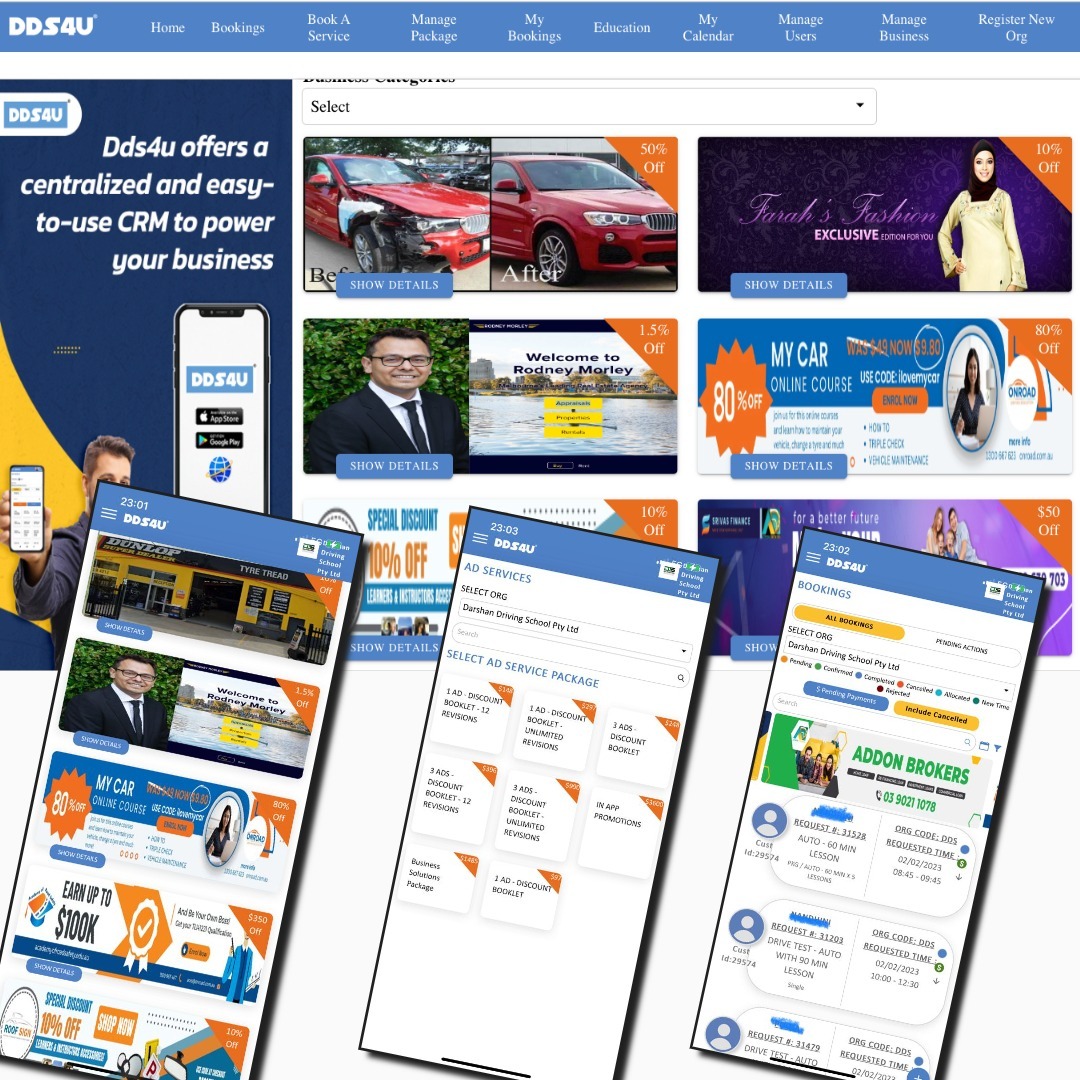The image features the interface of a business management application named DDS4U, with a primary blue-themed header displaying the logo "DDS4U" and several menu options. These options include: Homes, Booking, Rent-a-Service, Manage Packing, Package, My Booking, Education, My Calendar, Manage Users, Manage Business, and Register New Org.

Beneath the header, there is an informational section that describes DDS4U as offering a "centralized and easy-to-use CRM to power your business." The main content area displays a smartphone screen showcasing various promotional offers and deals items within the app.

1. **Red Damaged Car Promo**: A before-and-after image of a red car showing damage and then the repaired condition, with a message that says, "Welcome to Rodney Morley, 15% off," accompanied by a "Show Detail" button.
2. **Fashion Exclusive Promo**: An image of a woman wearing a white dress and a black hijab with a banner stating "Fairest Fashion Exclusive, 10% off," and a "Show Detail" button.
3. **Car Service Promo**: A picture of a lady sitting at a desk titled "My Car Chorus," offering "80% off" displayed in the right-hand corner and a "Show Detail" button.

The app interface is consistently displayed throughout, highlighting its user-friendly layout and various promotional offers to engage users.